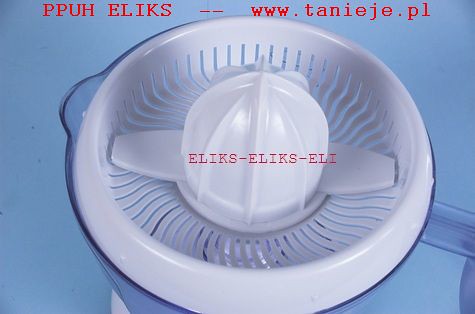The image depicts a manual juicer made of plastic, designed for squeezing citrus fruits by hand. The juicer consists of a white plastic top with multiple slits extending from the outer edge to the center, forming an open grating area. At the center, there is a dome-shaped, bulbous part with ridges, which appears to be used for pressing and rotating fruit such as oranges or lemons to extract juice. This dome is accompanied by two plastic blades resembling propellers, likely serving to prevent seeds from passing through the slits.

Below the juicing component, the device is connected to a transparent plastic bowl divided into small sections at the back. This bowl sits atop a blue base, which features a small groove in the bottom right corner. To the left, you can see part of a spout, and on the right, a rectangular handle attaches to the container, further suggesting it functions as a pitcher for collecting juice. 

The background of the image is blue, adorned with red text including the brand name "E-L-I-K-S E-L-I-K-S E-L-I" in the middle. The top of the image displays the text "P-P-U-H E-L-I-K-S W-W-W dot T-A-N-I-E J-E dot P-L" in red.